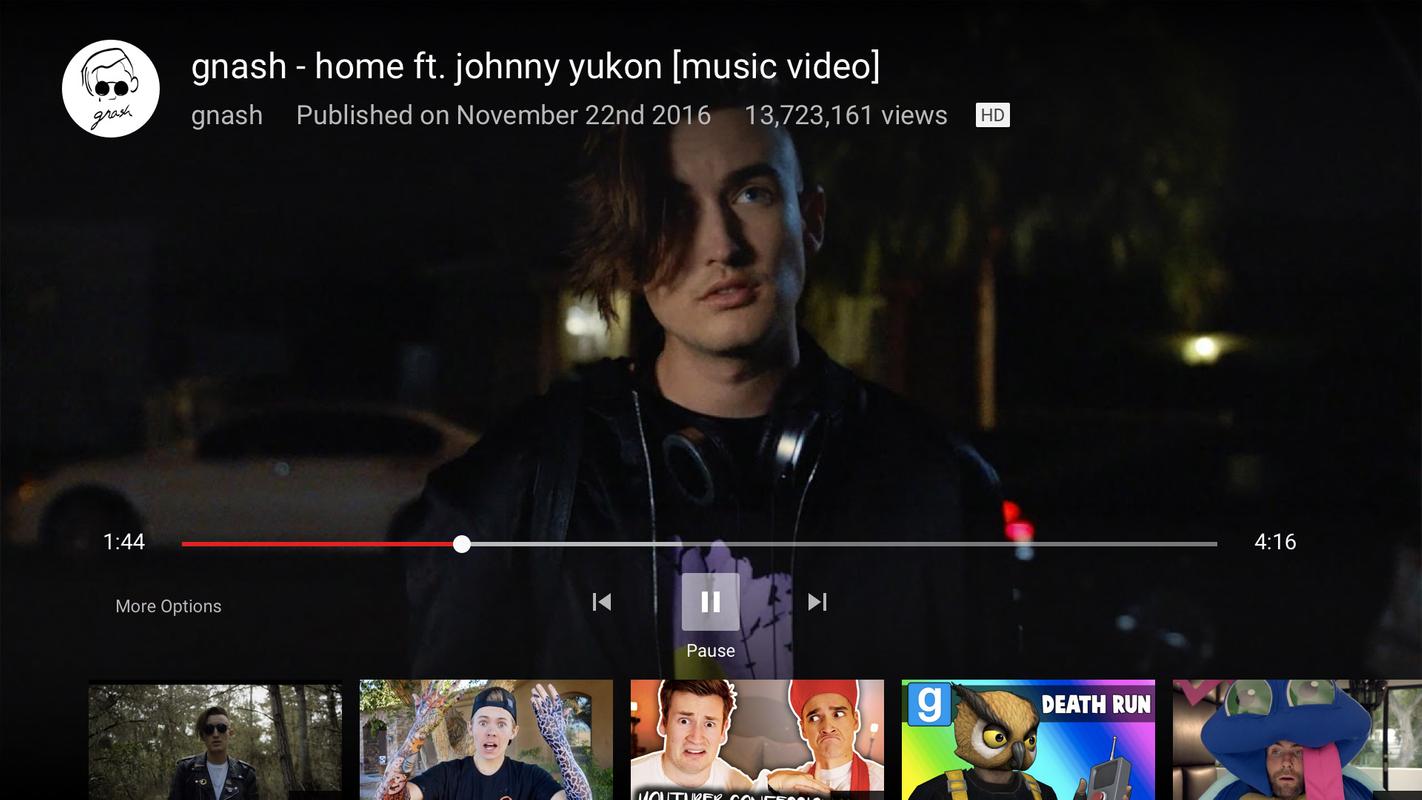Here is a cleaned-up and detailed caption for the image:

---

The screenshot captures a video in progress. In the upper left-hand corner, a white circle features the silhouette of a boy wearing round sunglasses. To its right, the video title reads "Nash - Home (feat. Johnny Ugon)" followed by a note stating it's a "Music Video." Just below, the text specifies "Nash - Published on November 22, 2016" along with the view count "13,723,161 views." Further, the HD definition indicator is displayed. The video is paused at 1 minute and 44 seconds, showing a male figure wearing headphones and a black coat. His hair is long and styled to swoosh to the right.

---